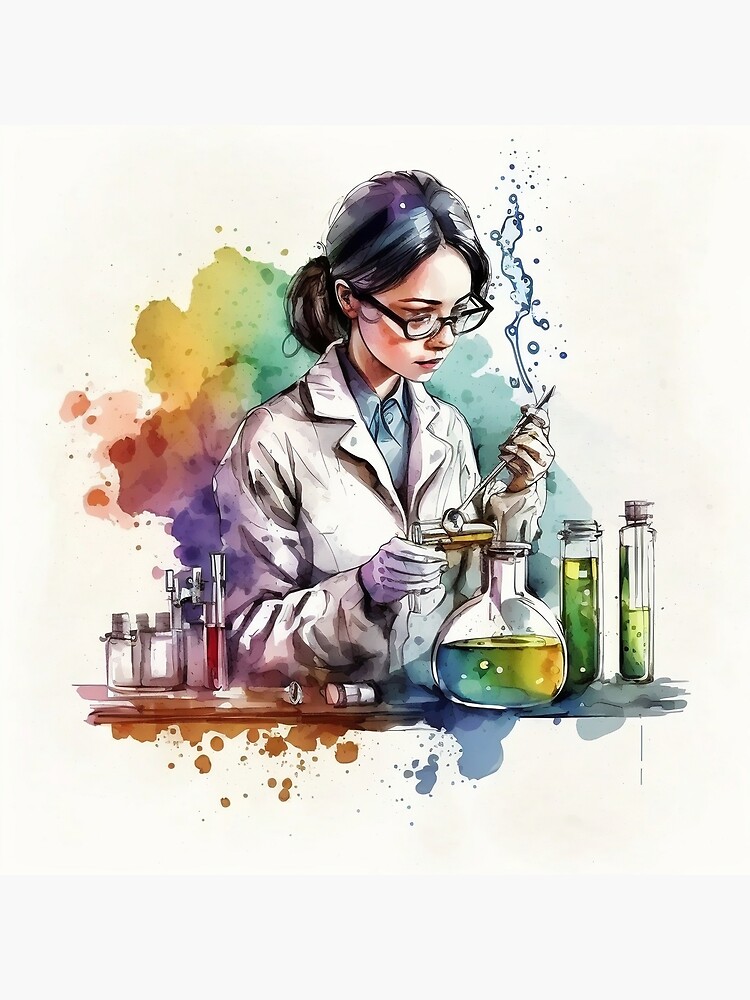The image portrays a detailed and colorful illustration of a young female scientist in her 20s, meticulously working in a laboratory. She is seen wearing a white lab coat over a light blue shirt, with purple vinyl gloves covering her hands. Her dark hair, streaked with purple, is neatly tied back in a ponytail. She peers through her black horn-rimmed glasses, concentrating on a series of beakers on the lab bench in front of her.

The scientist is depicted holding a tool in her left hand over an indistinct object, while in her right hand she elevates a test tube. The laboratory setup features three prominent beakers, all containing a greenish-yellow substance. Two of these beakers are long and narrow, standing upright on the table, while the third has a wide, round base and an open neck, reminiscent of a Florence flask.

The backdrop is a vibrant mix of watercolor hues, including green, yellow, purple, and red, which blend into the white background, adding a dynamic and artistic element to the scene. The colorful stains intriguingly extend to the desk in front of her, enhancing the visual appeal of the laboratory environment. The overall composition vividly captures the focused and intricate nature of scientific work.